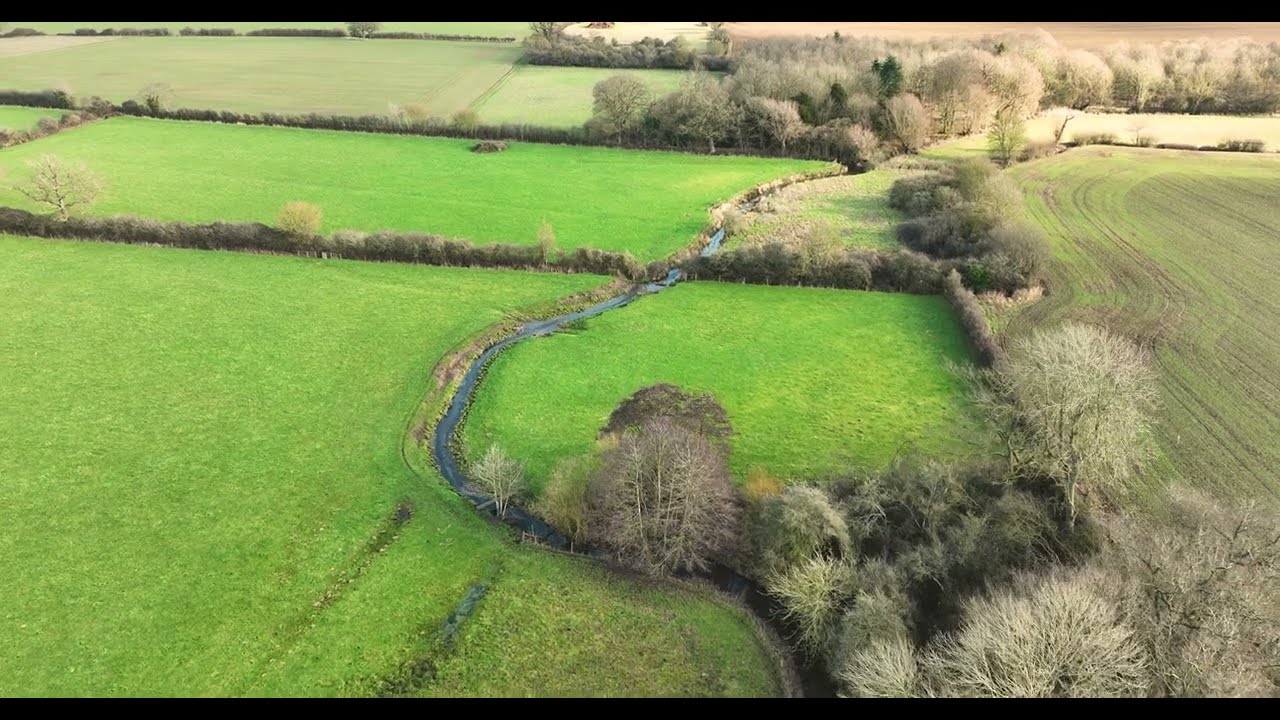The image depicts an aerial view of a farm field with a prominent stream running through the landscape. The stream, with its blue waters, starts roughly in the middle of the image, meandering in an S-shape towards the top right corner. The fields are sectioned off by a combination of trees, bushes, and what might be hedges. On the right-hand side, a dry, tilled field with noticeable lines contrasts with the very green grass on the left. In the foreground, deeper streaks in the grass, possibly from vehicle tracks or furrowing, extend from the stream down to the bottom edge of the image. The scene is framed by thin black borders at the top and bottom, giving a cropped appearance. Various trees around the field appear to be losing their leaves, introducing a grey hue, especially in the background, where their presence increases.